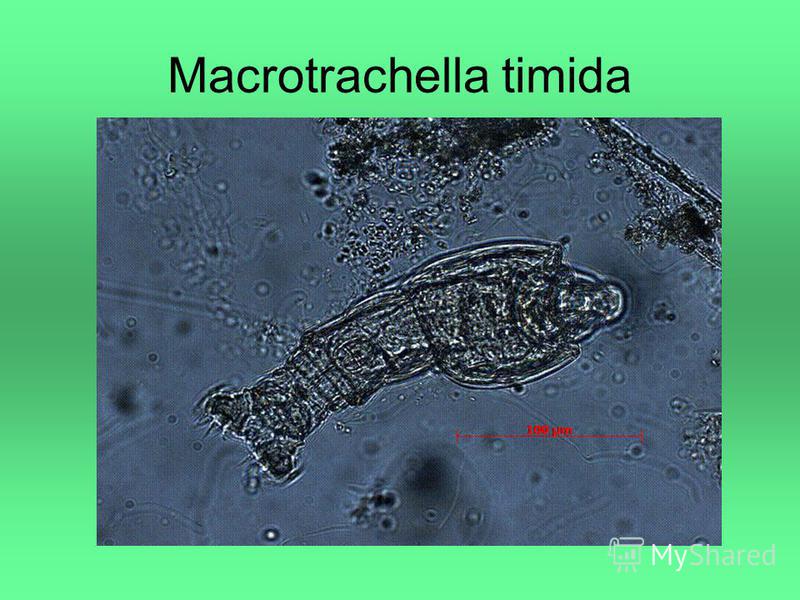This is a detailed color image, part of an informational slide or PowerPoint presentation, showcasing the microorganism Macrotrachella timida, prominently displayed at the center. The photograph, predominantly gray on a dark bluish-gray background with black and white tones, seems to be taken through a microscope. It features semi-transparent circles and lines, giving a layered, see-through effect to the scene. In the main section of the image, running from the middle left to the bottom corner and towards the middle right, lies the magnified organism. It has a detailed, intricate structure resembling a lobster-like creature without legs, more akin to a worm with a tail. There are spiky, arm-like appendages on either side, leading to a head and torso region. The photograph is encased in a light green border with black text at the top that reads "MACROTRACHELLA TIMIDA" and white text in the bottom right corner stating "MY SHARED." A small red legend or scale, which mentions the measurement "100," is also present, though the specific units are unreadable. The overall appearance is reminiscent of a Roman statue bent over, emphasizing the creature's unique and striking morphology.